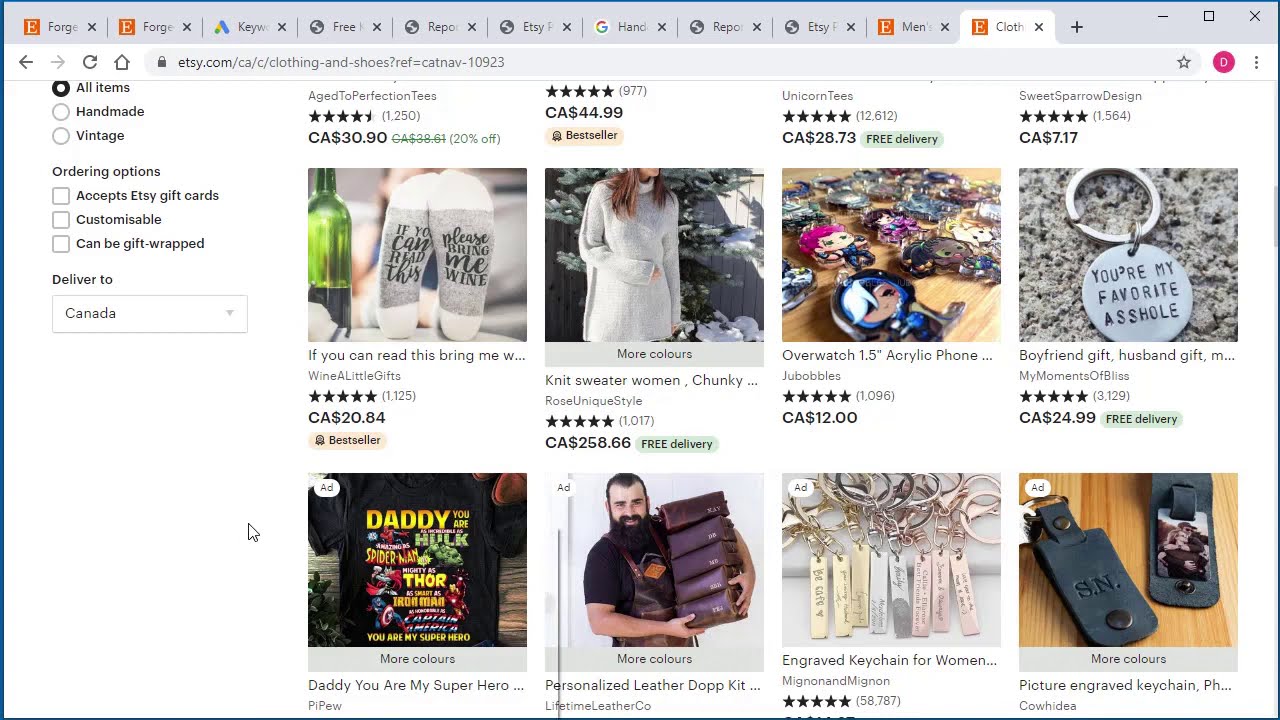Screenshot of an Etsy page displaying numerous open tabs at the top, with a grey bar spanning across and one highlighted white tab. The windows controls (line, square, and X) are located in the upper right corner. Below, the browser's navigation buttons (a highlighted back arrow, a greyed-out forward arrow, refresh, and home button) and a web address bar displaying 'Etsy.com' are visible.

On the left side of the page, a detailed list reads: "All items handmade, vintage," followed by "Ordering options," "Accepts Etsy gift cards," "Customizable," "Can be gift wrapped," and "Delivered to: Canada."

The main section of the page showcases various items for sale, described by the observer as "basically junk." Each item is priced in Canadian dollars, indicated by "CA$" preceding the amounts. Among the items, a particular favorite stands out on the far right of the first/second row: a grey keychain with the inscription "You're my favorite asshole" written in black.